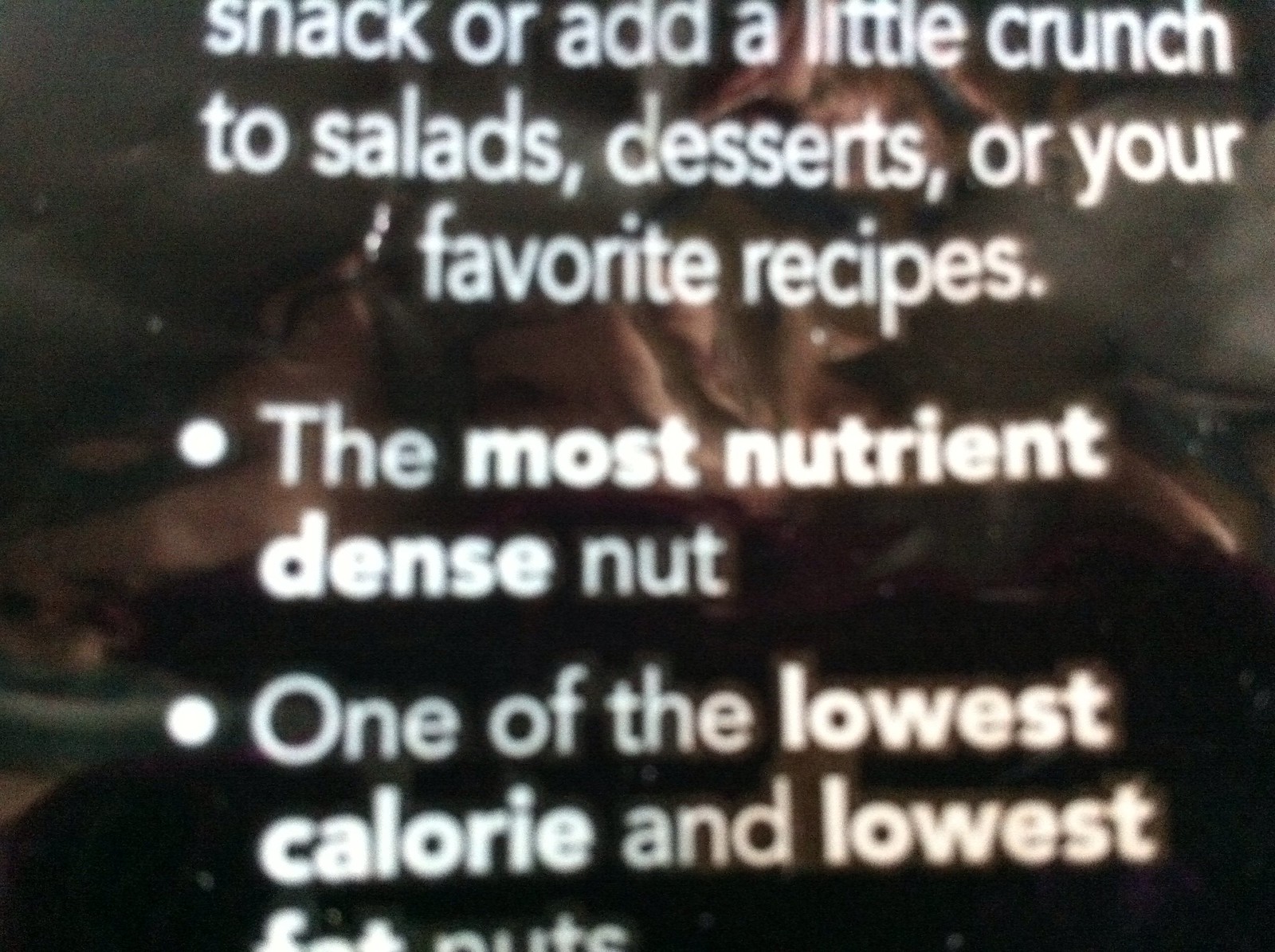This extreme close-up image captures a detailed portion of a product label or webpage, focusing on the descriptive text about certain nuts. The background features an indistinct brown area, adding to the mystery of the setting.

At the top of the image, white text reads: "Snack or add a little crunch to salads, desserts, or your favorite recipes." Below this, a small white dot precedes more text: "The most nutrient-dense nut." Another dot beneath this is followed by the words: "One of the lowest calorie and lowest fat nuts." While no nuts are visible in this close-up, the emphasis on nutritional benefits clearly indicates that the content is related to nuts. The close-up nature of the photo makes it difficult to discern additional details about the package or webpage background.